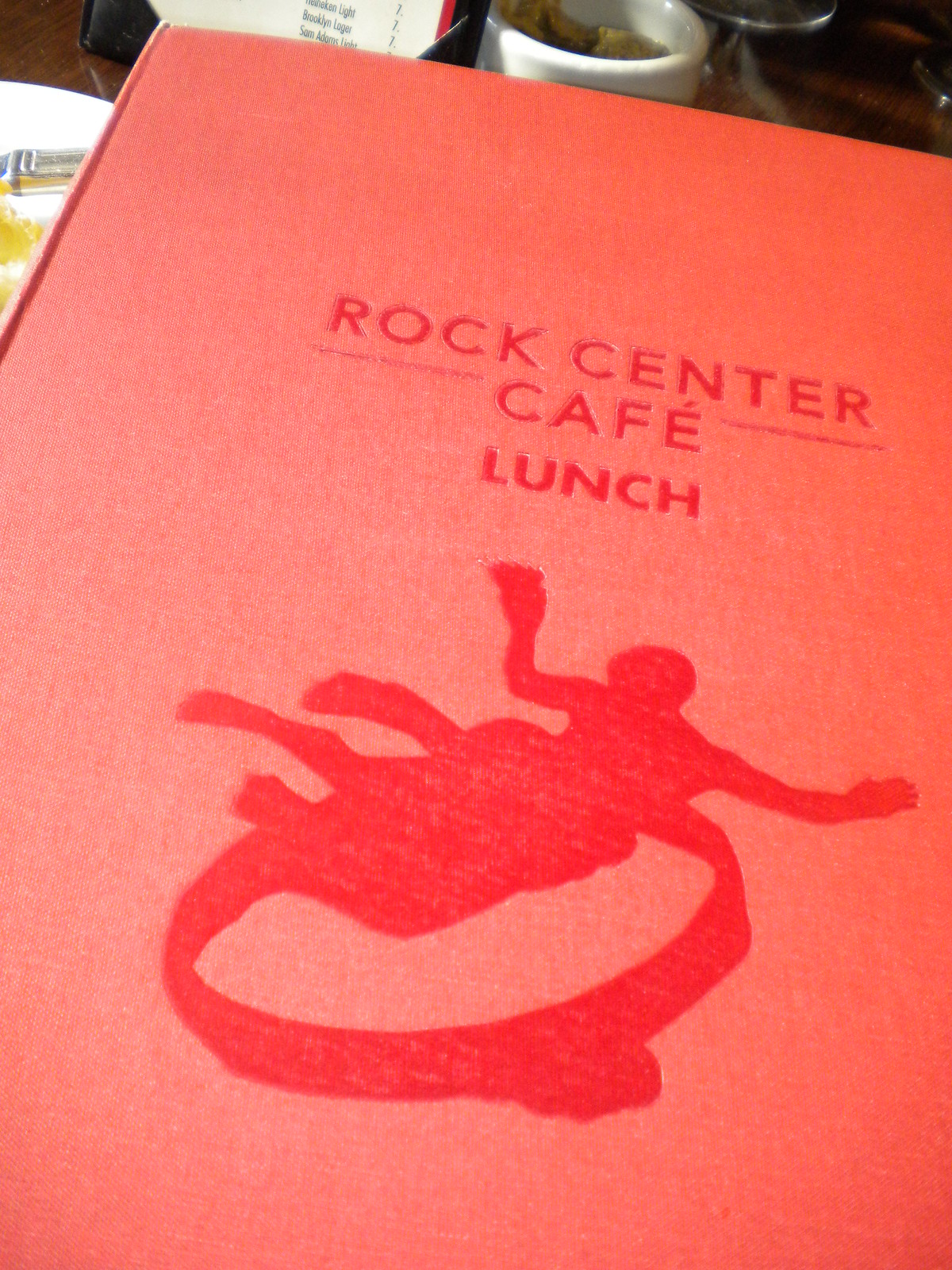The image features a close-up view of a menu cover from the Rock Center Cafe, likely situated in Rockefeller Center, New York City. The menu cover is a vibrant red, adorned with the indented text "Rock Center Cafe Lunch," which is also in red but stands out due to the indentation. Below the text "Cafe," there's a small logo in a darker shade of red, depicting what appears to be a human figure with multiple legs or possibly a man entangled in a ring. 

The menu lies on a table, partially surrounded by additional items such as a coffee cup, other menus, dishes, and condiment bowls, which are only partially visible along the edges of the photograph. The close-up nature of the image primarily highlights the detailed design and color of the menu cover.